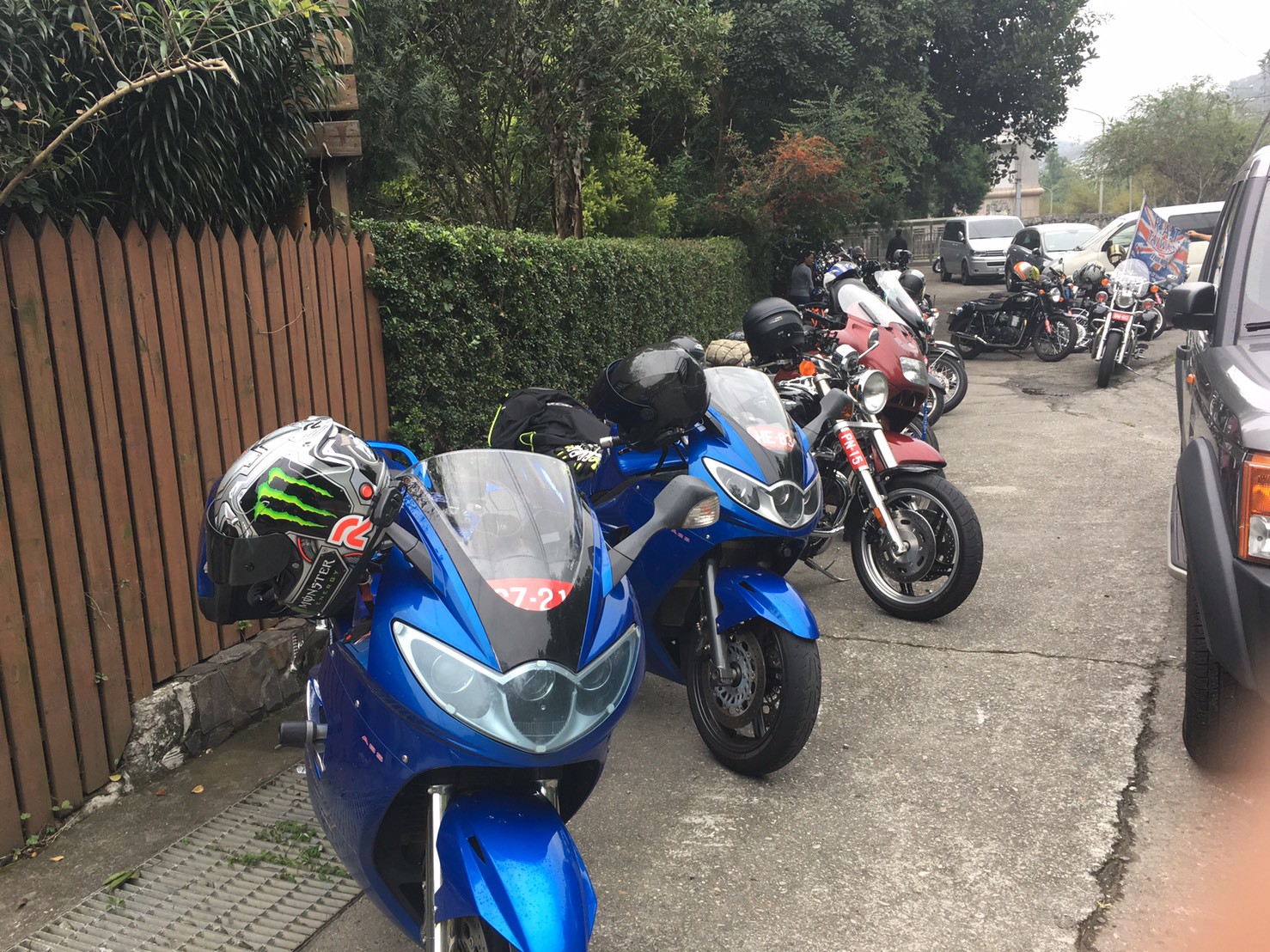This photo captures a tranquil neighborhood sidewalk scene dominated by a lineup of vibrant motorcycles and cars. In the foreground, a tall, brown picket fence partially covered in green vines runs parallel to a green hedge, both standing about five or six feet tall. A series of six motorcycles is prominently displayed along the sidewalk, four of which are parked at an angle in a neat row. The first two motorcycles boast a striking cobalt blue finish, followed by a vivid red bike and a sleek silver one. Further behind, a black and gold motorcycle faces the camera while another with red trim appears in the distant background, accompanied by a flag bearing a version of the British flag. Notably, several of the bikes feature helmets casually draped on the handlebars, including a distinctive light gray helmet emblazoned with the green Monster Energy drink logo.

Adjacent to the sidewalk, a road runs parallel, where four cars in varying shades of silver are parked, including a noticeable gray Jeep and a white van. The scene is set against a lush backdrop of tall trees, with faint suggestions of mountains peeking through the foliage. Completing the composition is a glimpse of a building corner and a sliver of blue sky overhead, adding depth to this serene suburban tableau.